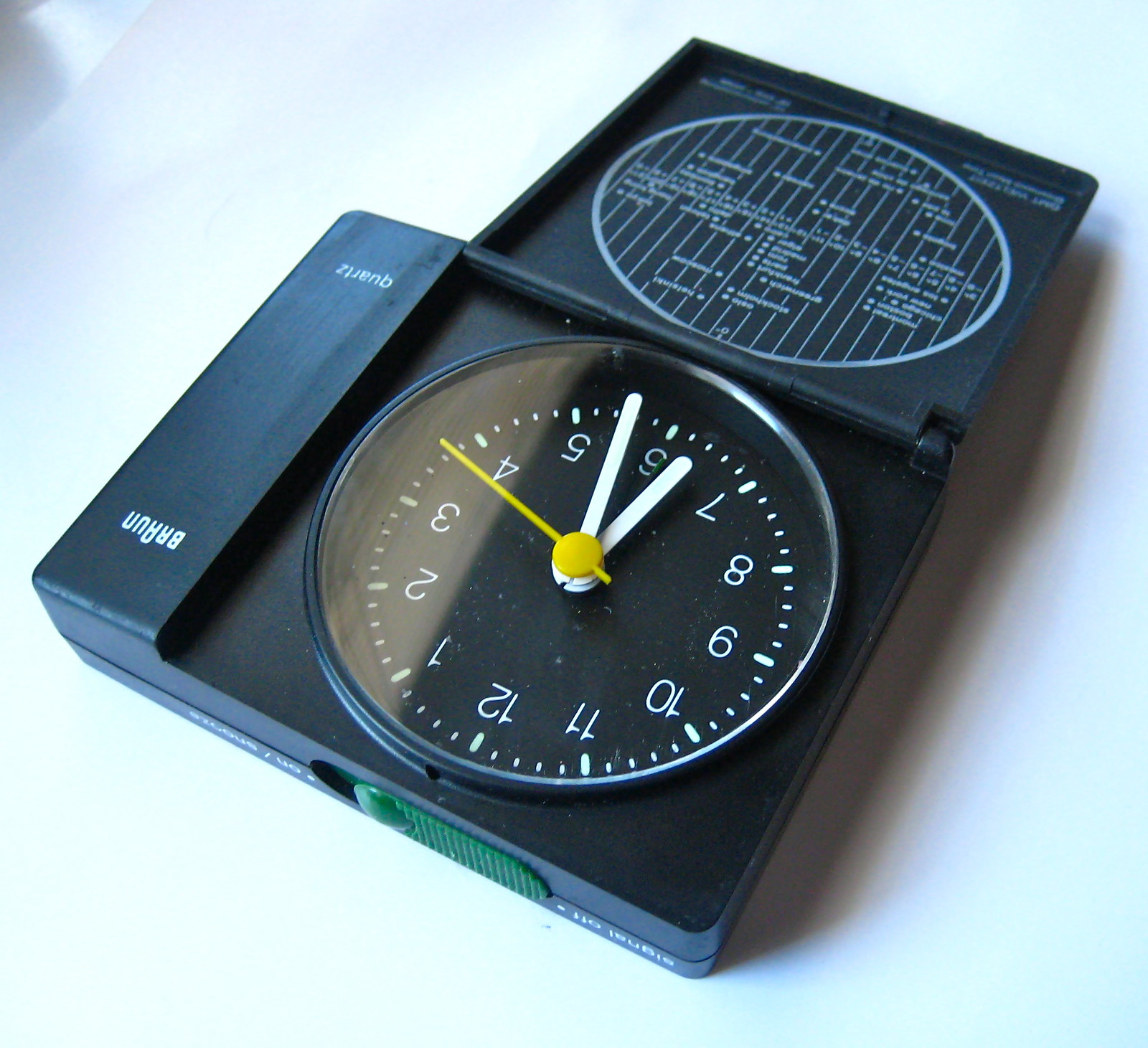This image features a unique clock encased within a transparent box. The clock, made by Brahm, is a quartz timepiece, distinguishable by its precise hour, minute, and second hands. The clock's sleek, circular face is black, contrasting sharply with its white numerals and markings. The time displayed is approximately 6:28. The transparent box serves as an unconventional yet intriguing cover for the clock, providing a clear view of its elegant design. This striking presentation raises questions about the purpose and appeal of encasing a clock in a box, as opposed to the convenience of a wristwatch.